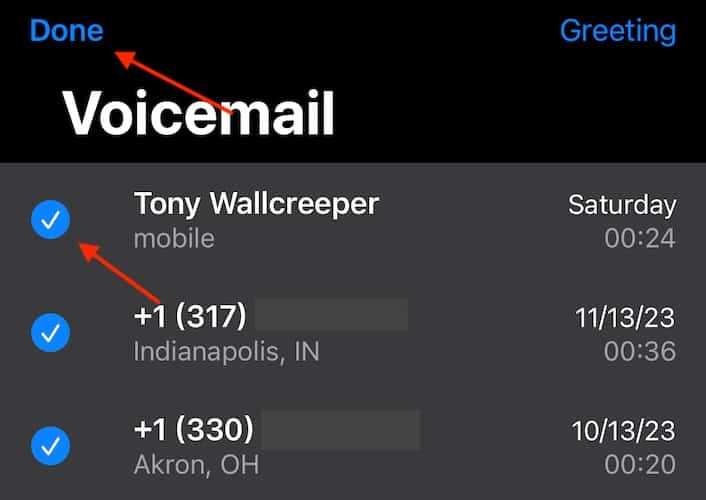Screenshot of a Voicemail Page on a Phone: 

The top bar of the screen is black with the word "Voicemail" prominently displayed in large white letters. Adjacent to this, on the left, there's a red arrow pointing to blue text that says "Done," indicating the option to finish viewing voicemails. On the right side of the top bar, there is blue text labeled "Greeting."

Below the "Voicemail" title, the screen displays three entries for phone calls and voicemails. 

1. The first entry is from "Tony Wall Creeper"; the voicemail was received on Saturday and is 24 seconds long, made from a mobile phone. A blue circle with a white checkmark is positioned to the left of his name.

2. Following this, there is a partial phone number from Indianapolis, Indiana, with the visible segment being "1" and the area code "317." This voicemail was left on November 13, 2023, and lasts 36 seconds.

3. The final entry shows a call from Akron, Ohio, with a partial number starting "1" and area code "330." This voicemail was left on October 13, 2023, and has a duration of 20 seconds.

Each voicemail entry provides detailed information about the origin, date, and length of the message, ensuring the user knows the essential details at a glance.